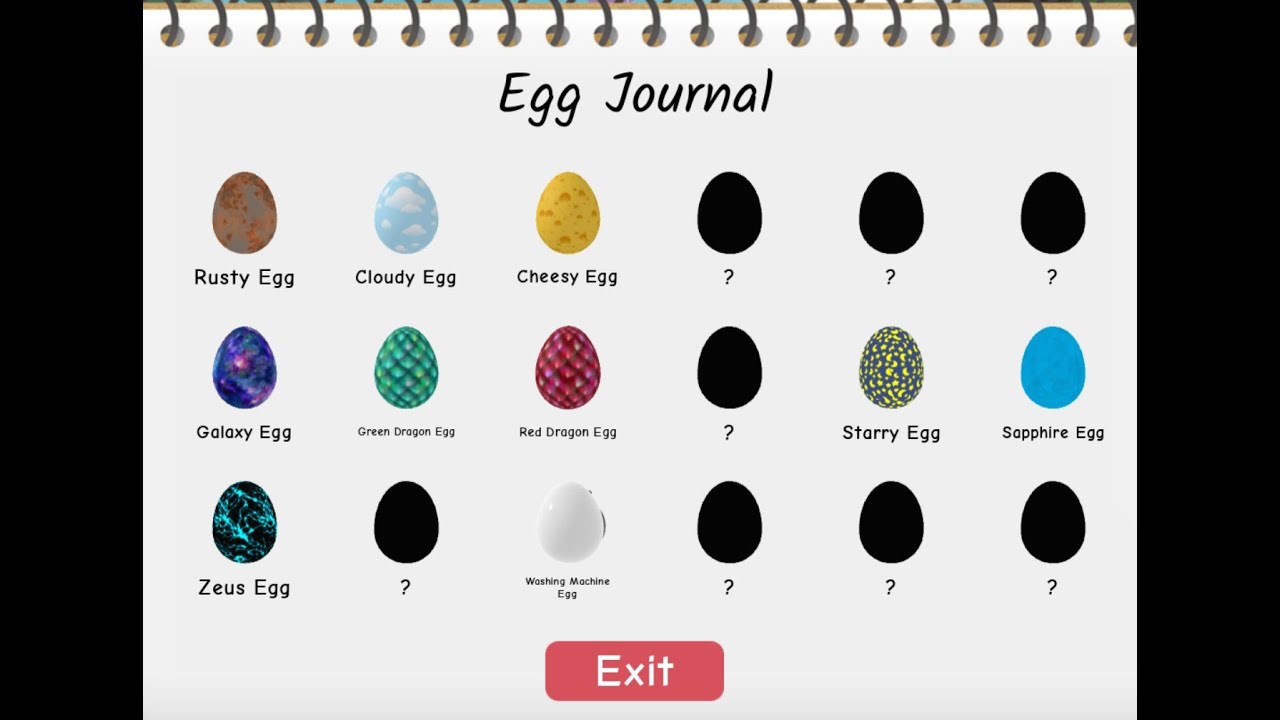The digital image showcases a vibrant illustration of a cartoon-style notebook, presented in a whimsical and playful manner. The notebook features a predominantly white background with a subtle gradient transitioning to light gray at the bottom, and it is bound with spiral rings at the top. At the very top of the paper, bold black comic-style text reads "Egg Journal."

Beneath this heading, an array of intricately designed eggs is displayed in a methodical grid format consisting of six columns and three rows:

- **First Column:** 
  - Top Row: "Rusty Egg," a brownish-hued egg.
  - Middle Row: "Galaxy Egg," adorned with a nebula-like purple design.
  - Bottom Row: "Zeus Egg," black with aqua blue splashes.

- **Second Column:**
  - Top Row: "Cloudy Egg," featuring a blue base with white cloud patterns.
  - Middle Row: "Green Dragon Egg," covered in green scales.
  - Bottom Row: "Question Mark Egg," a mysterious, fully black egg with a question mark.

- **Third Column:**
  - Top Row: "Cheesy Egg," showcasing a yellow cheese pattern.
  - Middle Row: "Red Dragon Egg," depicted with red scales.
  - Bottom Row: "Washing Machine Egg," shiny and white with a polished look. 

- **Fourth Column:**
  - Top Row: "Question Mark Egg," another enigmatic black egg with a question mark.
  - Middle Row: "Question Mark Egg," similar to the ones above.
  - Bottom Row: "Question Mark Egg."

- **Fifth Column:**
  - Top Row: "Question Mark Egg," yet another black egg with a question mark.
  - Middle Row: "Starry Egg," displaying a dark green background with yellow specks.
  - Bottom Row: "Question Mark Egg."

- **Sixth Column:**
  - Top Row: "Question Mark Egg," a consistent black egg with a question mark.
  - Middle Row: "Sapphire Egg," marbled in a light blue color.
  - Bottom Row: "Question Mark Egg."

At the bottom of the notebook is a prominent red button labeled "Exit" in white text, offering a clear option to close or leave the page. This charming and detailed illustration invites viewers to immerse themselves in the quirky and engaging world of the "Egg Journal."